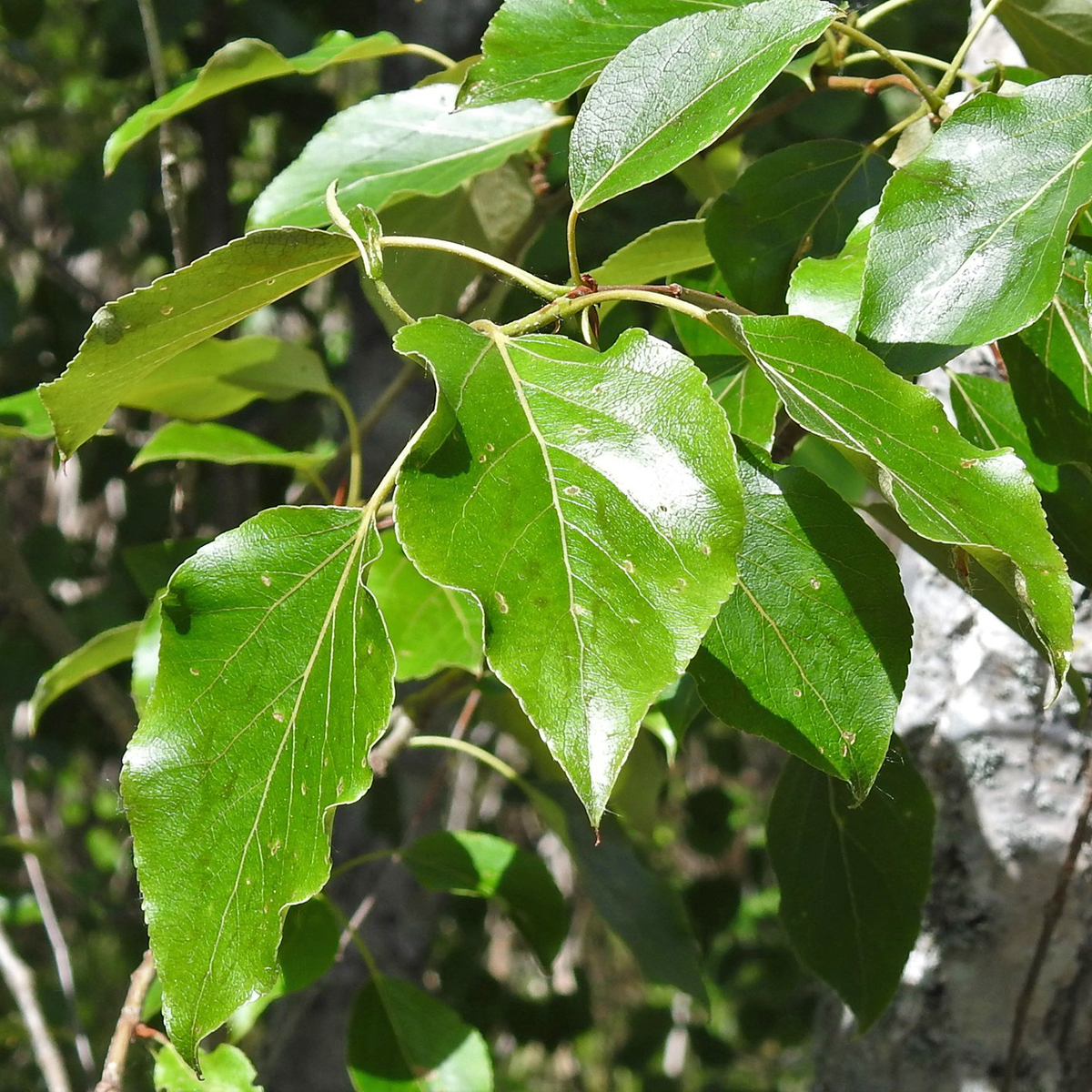This photorealistic image captures a close-up of a vibrant branch or plant emerging from a tree. The primary focus is on a cluster of roughly a dozen heart-shaped, bright green leaves, each characterized by striking white veins that radiate from the center to the edges. The leaves, shiny and slightly rounded at the tips, are oriented in various directions—some facing the viewer directly, while others point upwards or away. They are attached to a light green central branch that transitions to a brown hue as it recedes into the indistinct background. The background itself is a blurred blend of greens and browns, hinting at additional foliage and a forest floor composed of darker, earthy tones. Notably, some of the leaves show signs of minor damage, with tiny holes likely caused by unseen insects. Overall, the image offers a detailed and vivid portrayal of the main plant against the soft, natural backdrop of a lush, densely populated forest.